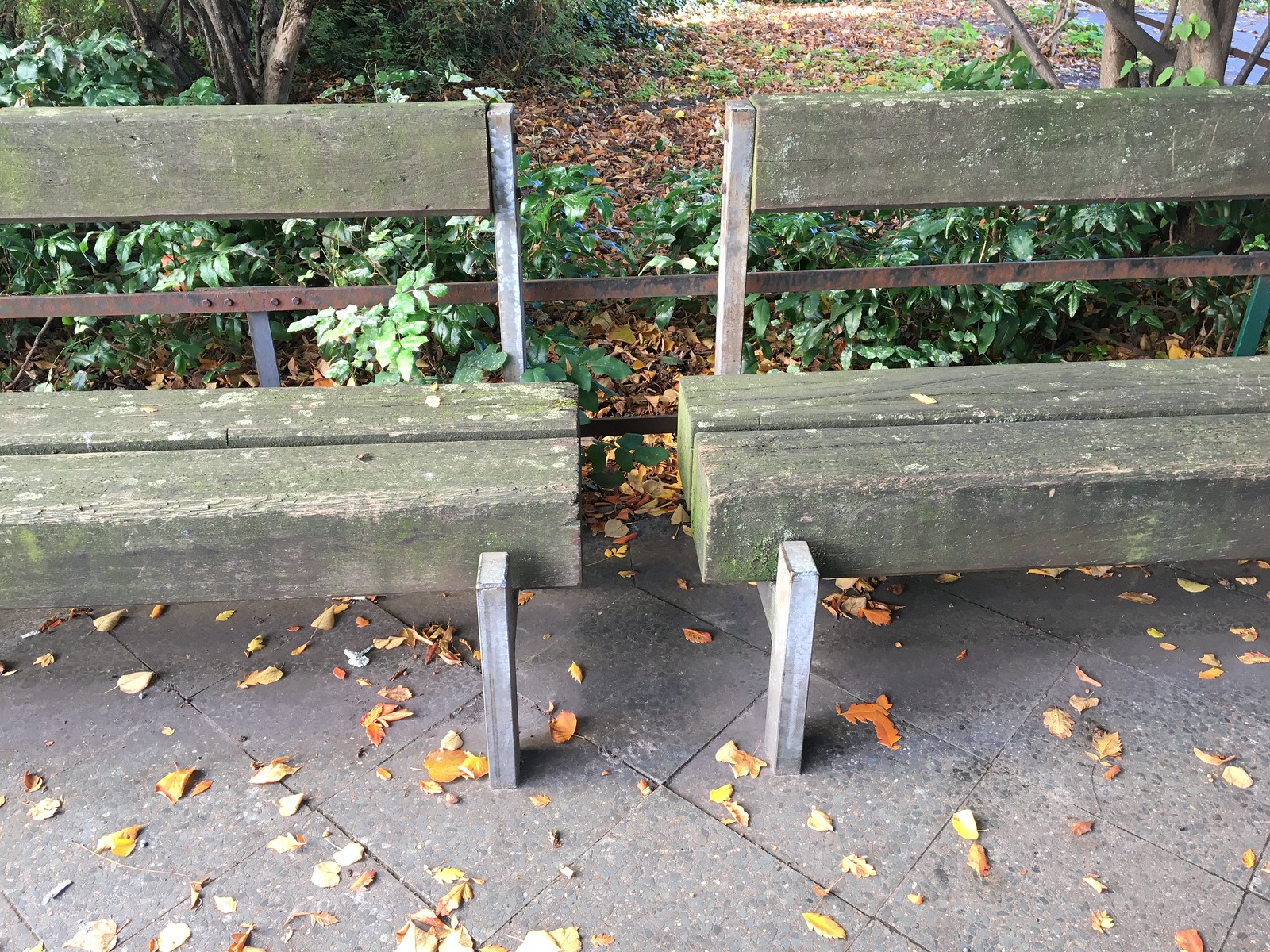This detailed image captures an outdoor area, potentially a park, featuring two weathered wooden benches set on a patio or stone walkway with silver-gray tiles. The aged benches, marked by green mold and scuffs, are supported by metal frameworks and show signs of prolonged exposure to the elements. The ground around the benches is covered with scattered dead leaves in orange, brown, and yellow hues. Surrounding the benches and lining the edges of the patio are rusty brown metal fences with visible bolts. Behind the benches, there is dense greenery, including bushes on both sides and trees emerging from the ground, providing partial views of a possible lake through the tree line on the top right. The concrete area where the benches are placed also shows a unique diamond pattern, contributing to the overall worn and rustic look of this serene natural setting.